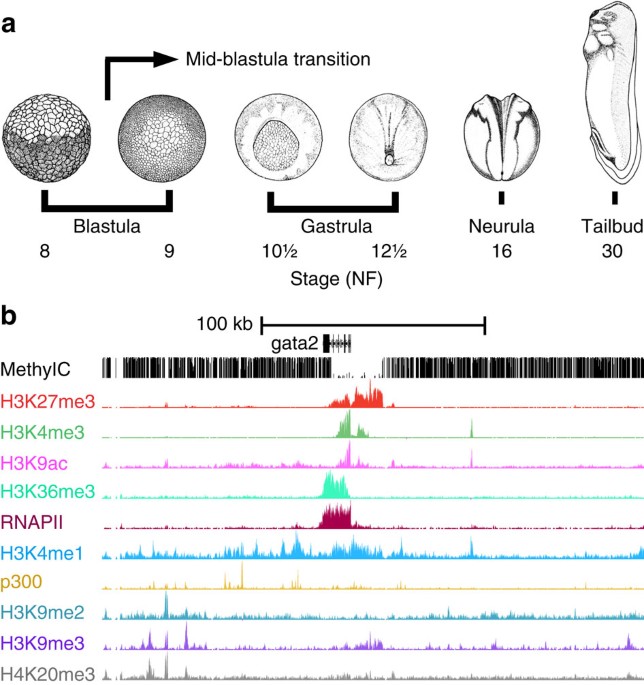The image is a detailed and technically complex chart illustrating embryonic development stages and related molecular data. At the top, the chart is divided into two parts, Part A featuring black-and-white drawings of embryonic stages, and Part B containing color-coded bar graphs representing various genetic markers. In Part A, the embryos are depicted progressing from the Blastula stage, where a group of cells develops, through the Gastrula stage with forming features and a sac-like structure, to the Neurula stage where these forms split more distinctly, and finally to the Tail Bud stage, which elongates into an animal-like shape. An arrow labeled "mid-Blastula transition" points to this critical developmental phase. 

Below these illustrations, Part B presents censored data in the form of various bar graphs with multiple rows (11 different categories) of information. Each row corresponds to specific genetic markers such as Methyl C, H3K27Me3, H3K4Me3, H3K9Ac, H3K36Me3, RNAP2, H3K4Me1, P300, H3K9Me2, H3K9Me3, and H4K20Me3. These graphs exhibit different patterns and colors (red, green, purple, blue, yellow), possibly indicating changes in gene expression or molecular activity during these embryonic stages. The overall composition of the image emphasizes a transition in cellular development and the corresponding genetic and molecular data associated with these stages.